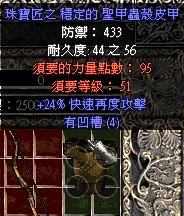This color image appears to be an advertisement, possibly a screenshot from a video game, featuring Chinese characters and prominent numerical values. The upper two-thirds of the image has a black background with various lines of text in different colors. 

At the top, a purple banner with Chinese characters is followed by a line of white characters, including a colon and the number 433. Subsequent lines continue with white Chinese characters interspersed with numbers, notably 44 and 56. Below these, there are rows of red text, with numbers 95 and 51. Two purple lines at the bottom of this section include a mention of "+24%".

The bottom third of the image is divided into three equal segments, each decorated with distinct designs. The left segment is maroon with gold squares, the middle segment features a gold, reflective, metallic leaf design with four circles resembling a lock, and the right segment contains an ornate piece of ironwork.

Overall, this visually striking image combines intricate design elements with textual information presented in vivid colors and various numeric values, creating a compelling and richly detailed advertisement.